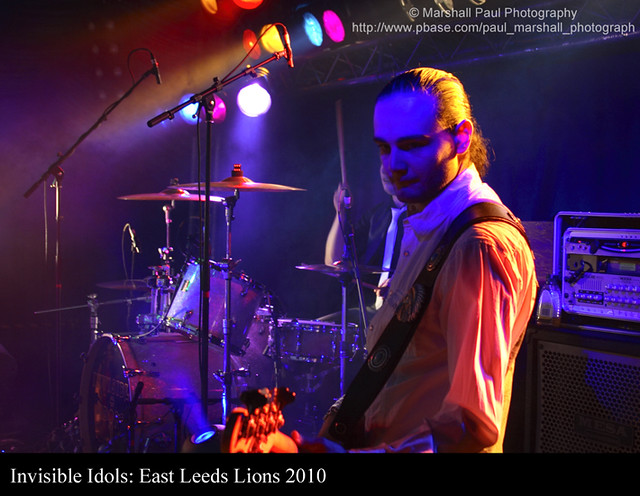The professionally shot photograph captures a dramatic and vivid moment from a 2010 concert by the band Invisible Idols, East Leeds Lions. The image is dominated by a guitar player, seen from the side, who is intensely focused on his instrument. He has long hair pulled back into a ponytail, and he wears a white button-up shirt that appears golden on his back due to the stage lighting, while the front remains dark with blue highlights. A guitar strap runs over his shoulder, and his left hand strums near the upper part of the guitar. The stage is enveloped in a dark ambiance, enhanced by smoky effects and a vibrant array of colored lights, including purple, blue, yellow, and red, casting dramatic hues. In the background, the drummer, dressed in a black jacket with a white shirt underneath, is partially visible amid the multi-colored lighting reflecting off the drum kit. The bottom left corner of the image notes the band's name and event details in white text: "Invisible Idols, East Leeds Lions, 2010." Additionally, the top right corner is inscribed with "Marshall Paul Photography," accompanied by the website http://www.pbase.com/paul-marshall-photograph. The overall effect is a visually striking portrayal of the dynamic concert atmosphere.